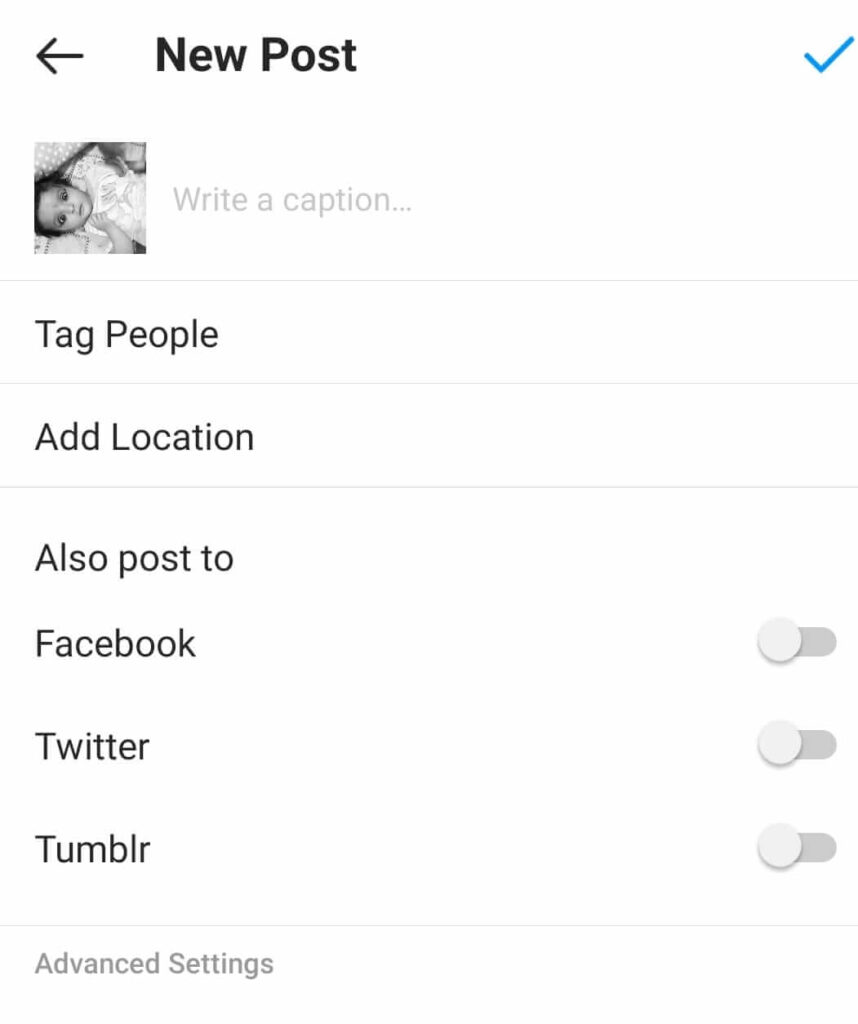The image captures a screenshot from a social media platform, likely Instagram, as it showcases the interface for creating a new post. The central feature of this screenshot is a black-and-white photograph of a little girl, possibly a toddler, with delicate facial features suggesting she is female. The platform prompts the user with "Write a caption" above the image area. Below, there are several options listed in a structured layout: "Tag People," "Add Location," and "Advanced Settings." Further down, there are toggles for cross-posting to other social media platforms, including Facebook, Twitter, and Tumblr, all of which are currently enabled, as indicated by the checked boxes next to each. The heading "New Post" is prominently displayed in bold, dark text at the top. On the top left corner, a back arrow icon is visible, and a blue checkmark is positioned at the very top, though it does not signify Twitter verification. The screenshot is set against a clean, white background, emphasizing the straightforward and user-friendly design of the interface.